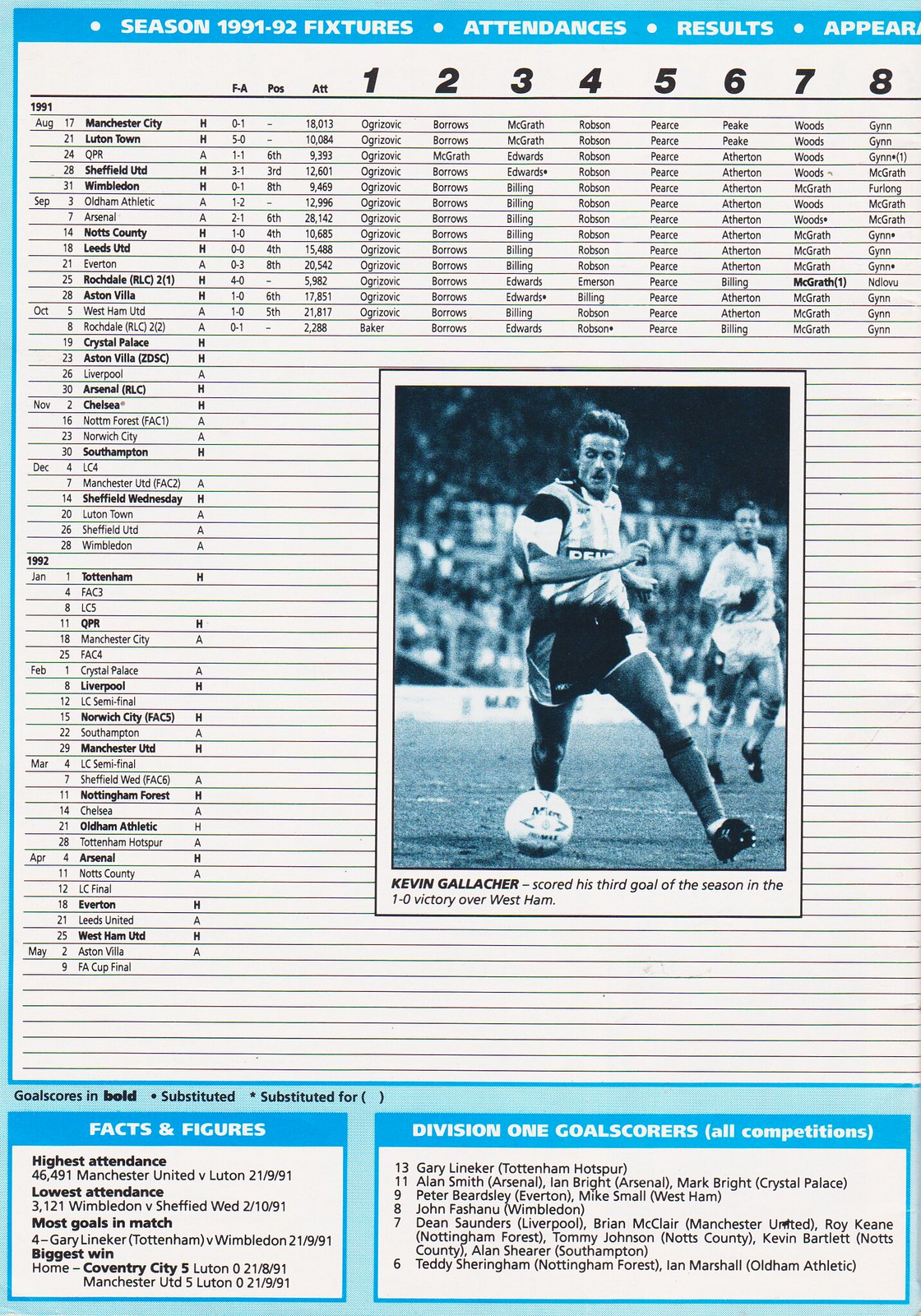The image is a detailed schedule for a soccer club from the 1991-92 season. At the top, a light blue banner spans the width of the page with the title "Season 1991-92 Fixtures, Attendances, Results, Appearances." On the far left, the schedule starts with "1991" and lists each month from August to December, and then continues with "1992" from January to May. Each month has five specific dates listed next to it, with the first match on August 17 against Manchester City and the final entry being the FA Cup Final on May 9. Each match entry is accompanied by a score or outcome indication and the team’s position after each game, along with attendance figures.

Across the top, heavy black numbers from 1 to 8 label columns with player names listed beneath each number. Just to the right center of the page, there is a black-and-white photograph of a soccer player running on the grass, focusing on the ball to his left. The player, who has black hair and is dressed in a jersey with black and white colors, mostly black shorts, and black shoes, is captured with his right foot poised beside the ball. Another player in a white jersey is running behind him, with the audience visible in the stadium background. The caption under the photo states, "Kevin Gallagher scored his third goal of the season in the 1-0 victory over West Ham."

At the very bottom of the image, there are two highlighted sections: "Facts and Figures" and "Division I Goal Scorers." The "Facts and Figures" section includes data on the highest and lowest attendances, most goals in a match, and the biggest win. The "Division I Goal Scorers" section lists top goal scorers in all competitions: Gary Lineker with 13 goals, Alan Smith with 11, Peter Beardsley with 9, John Fashanu with 8, Dean Saunders with 7, and Teddy Sheringham with 5, each cited with their respective cities in parentheses. The entire image features a distinct blue tint.